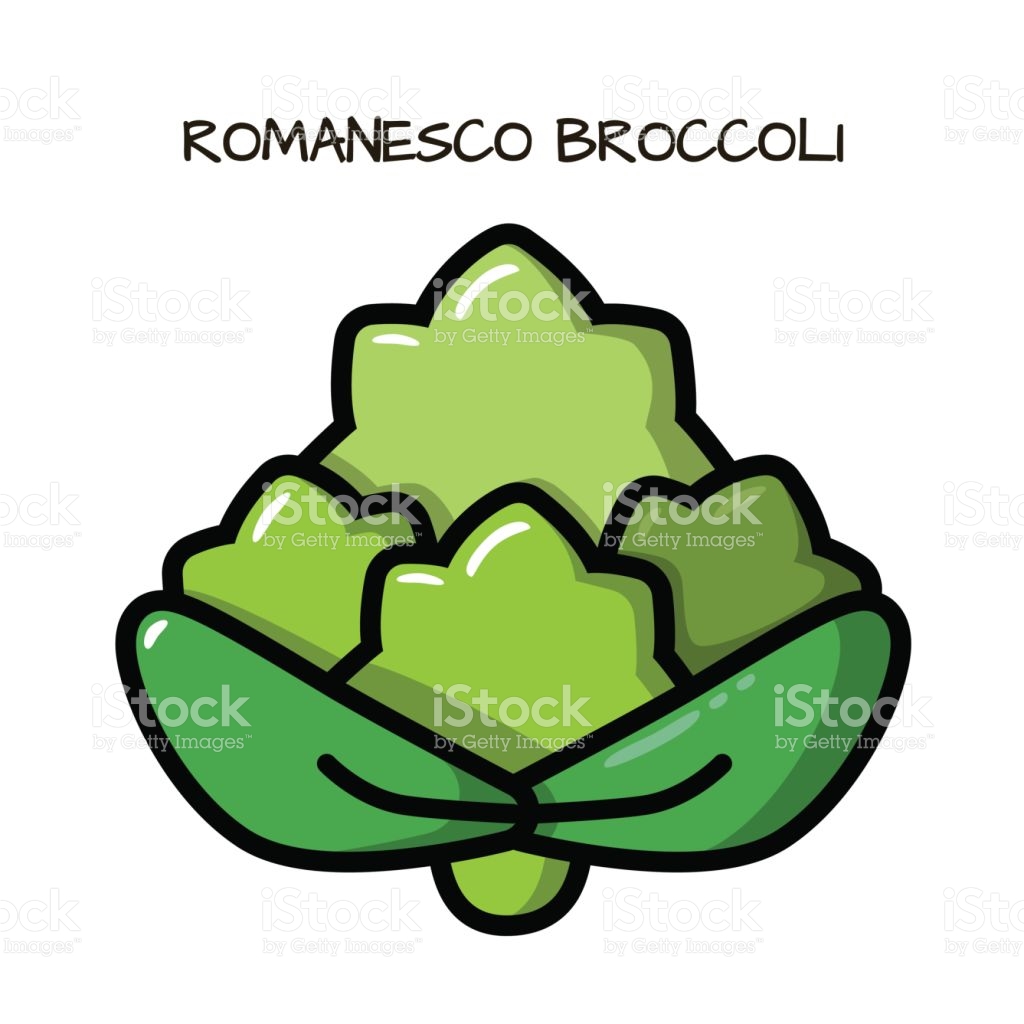This is a professional stock image cartoon drawing of Romanesco Broccoli with a prominent label at the top in black text that reads "Romanesco Broccoli." The image features a detailed hand-drawn depiction of the vegetable, exhibiting four pointy heads arranged in a star-like configuration. The broccoli heads are predominantly light green, transitioning to a darker green in the middle sections, with the stem and lower parts displaying the brightest green hue. The stalk is pale olive green, and there are two darker green leaves with distinct black lines running through them on either side of the stem.

The background of the image and the broccoli itself are covered with multiple "iStock by Getty Images" watermarks, indicating that this is a copyrighted stock image available for purchase. The overall color palette includes various shades of green along with black and white accents. There are no additional elements or people in the image, allowing the detailed illustration of the Romanesco Broccoli to occupy the central focus.